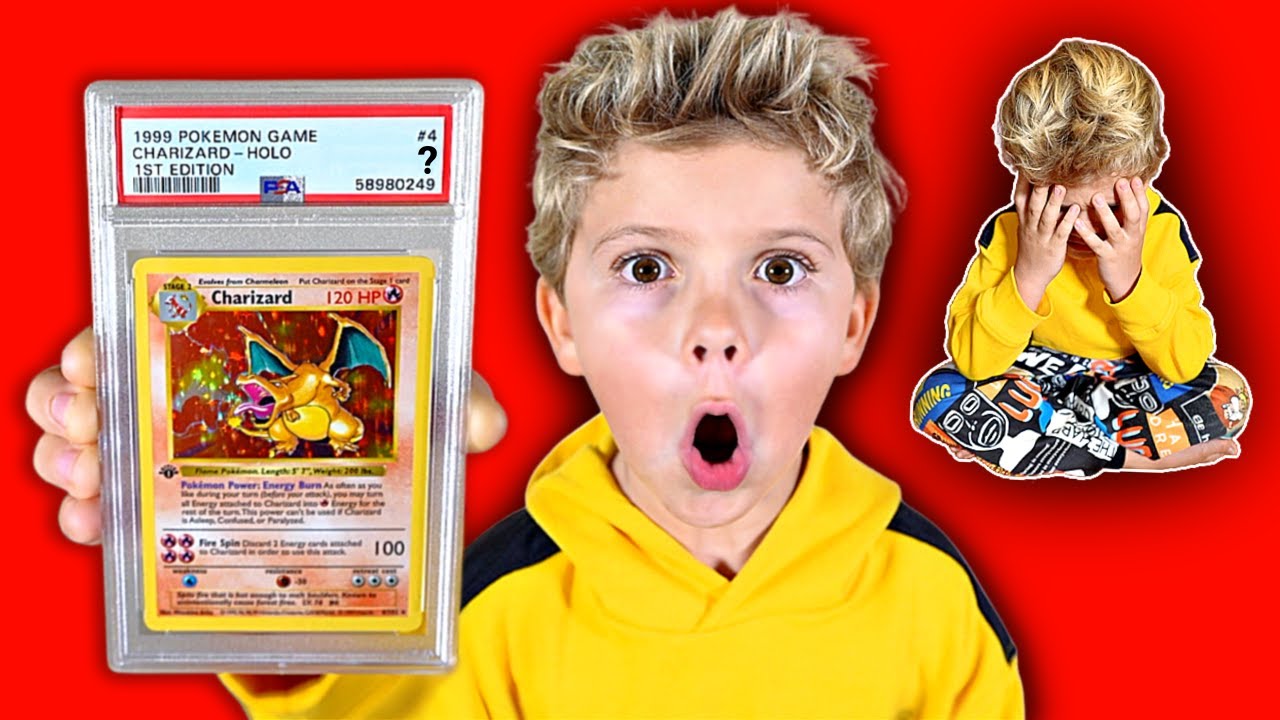In a vibrant red background typical of a YouTube thumbnail, a blonde-haired boy, appearing to be around seven or eight years old, is prominently featured. He wears a yellow jumper and displays a look of sheer astonishment on his face. His eyes are wide, and his mouth agape as he holds up a highly coveted 1999 Pokemon Game Charizard-Holo 1st Edition card, encased and in mint condition. The card, exhibiting 120 HP and shining with its holographic graphics, is clearly a prized collector's item. The text on the case emphasizes its rarity and value. In the upper right corner, a smaller image of the same boy is seen, sitting cross-legged with his head buried in his hands, looking distraught—perhaps dramatizing the emotional highs and lows of Pokemon card collecting. The dramatic drop shadows and bold red backdrop amplify the emotions, making the thumbnail visually striking and engaging.